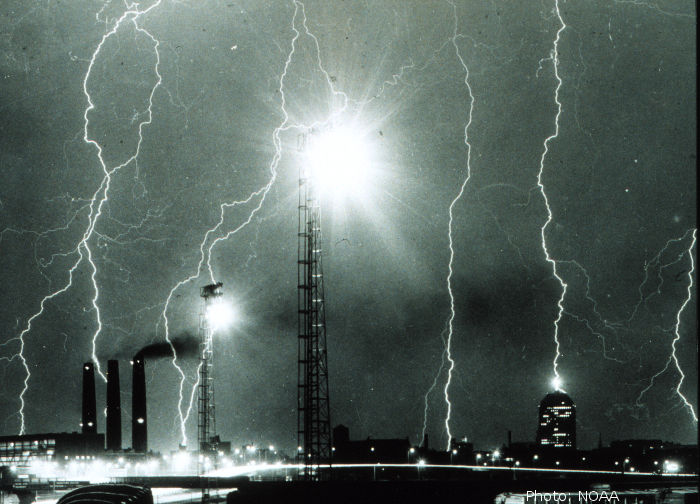This black and white photograph captures a dramatic nighttime scene in an industrialized area, dominated by a fierce lightning storm. Central to the composition is a tall metal scaffolding tower emitting a large beam of white light, flanked by a slightly smaller tower, which also has a glowing beacon, to its left. The sky above is dark and foreboding, punctuated by at least seven intense bolts of lightning, some appearing chained together. These lightning bolts strike various points across the cityscape in the background, targeting buildings, metal towers, and even the ground. Notably, a tall building on the right side of the image is illuminated from within, and a bolt of lightning dramatically connects to its rooftop. Toward the bottom left, three smokestacks rise, with one releasing smoke, suggesting the presence of a factory or power plant. Additionally, clusters of small white orbs scatter across the lower part of the photograph, adding to the image's chaotic energy. The intricate interplay of light, shadow, and industrial elements creates a riveting portrayal of nature's raw power amidst human development.